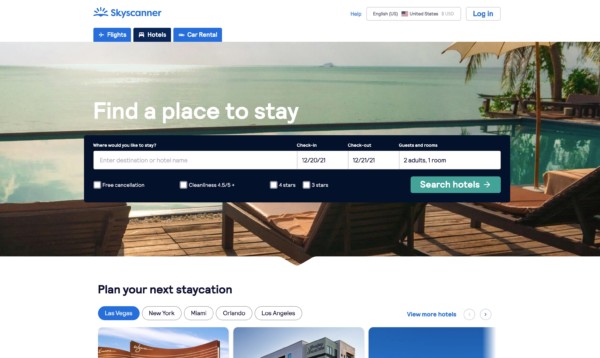A screenshot of the Skyscanner website in English, showcasing various travel-related options available for users. At the top, there is a login button. The main section features dynamic billboards with options for Flights, Hotels, and Car Rentals. An inviting vacation image displays a picturesque beach scene with crystal-clear waters and a sun umbrella, encouraging users to find a place to stay.

Prominently displayed is a blue square prompting users with the question, "Where would you like to stay?" Below this, fields for checking in and out are filled with the dates December 20, 2021, and December 15, 2021, respectively. The form indicates a selection for 2 adults and 1 room with a free cancellation option available. Filters for cleanliness ratings of 4 stars and 3 stars are visible along with a "Search Hotels" button.

The page also showcases wooden boards and chairs with a phrase, "Plan your next vacation," and lists popular destinations such as Las Vegas, New York, Miami, Orlando, and Los Angeles. Carousel arrows suggest that there are additional hotel options to explore. Overhead, a bright blue sky dominates the background, emphasizing the theme of leisure and travel. In the center, a striking building accentuates the professional layout while the caption, "A few more hotels," implies a wide range of accommodation choices.